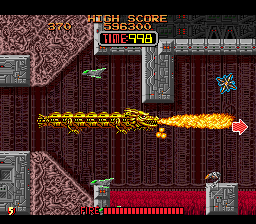This image is a detailed screenshot of an arcade-style video game set within a castle environment featuring prominent lava flows at the bottom of the screen. At the center, a long, gold dragon extends from left to right, breathing fire towards the right side. The fire is accompanied by an arrow and a blue and yellow star emerging from it. At the top of the screen, a high score of 596,300 is displayed alongside a timer reading 998. The bottom of the screen showcases a silver square base amidst red bricks and a label that reads "fire." The scene is also dotted with a bird flying across, adding to the dynamic visual elements.